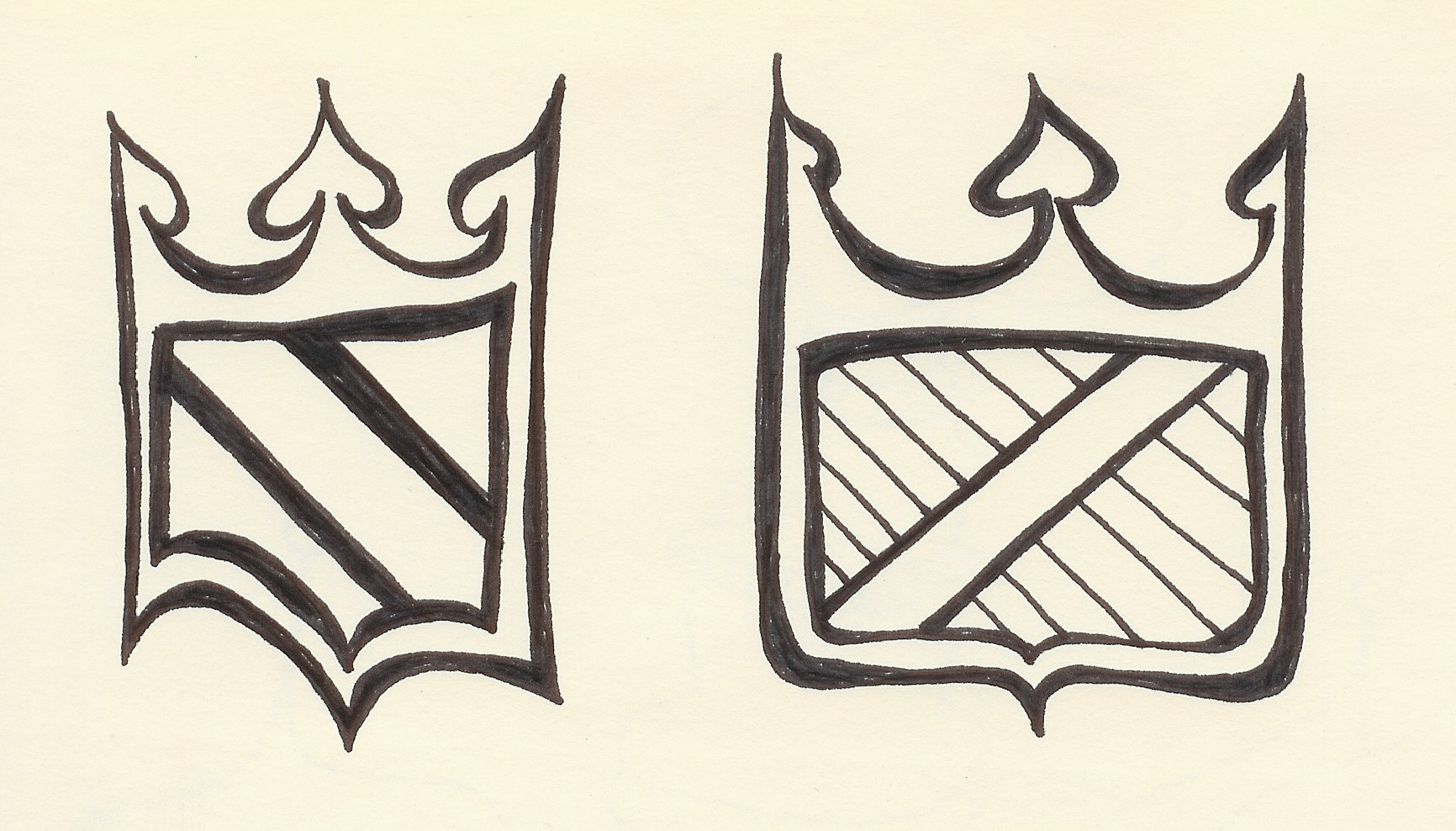This image features a detailed drawing of two shields set against a background with a pinkish-white, almost yellowish hue, reminiscent of aged paper. Both shields are rendered in black marker, emphasizing a stark black-and-white contrast. The shield on the right is notably wider than the one on the left but shares a similar intricate design.

Each shield top features a central spade shape, flanked by two half-spades on either side, creating a symmetrical and regal appearance. The shield on the left has a central design of two diagonal black stripes running from the top left to the bottom right. In contrast, the shield on the right features an intricate pattern within a rectangular center area, displaying multiple diagonal lines overlaid with one prominent diagonal stripe running in the opposite direction. The artwork showcases a combination of repeated motifs and unique details, suggesting a symbolic or heraldic significance.